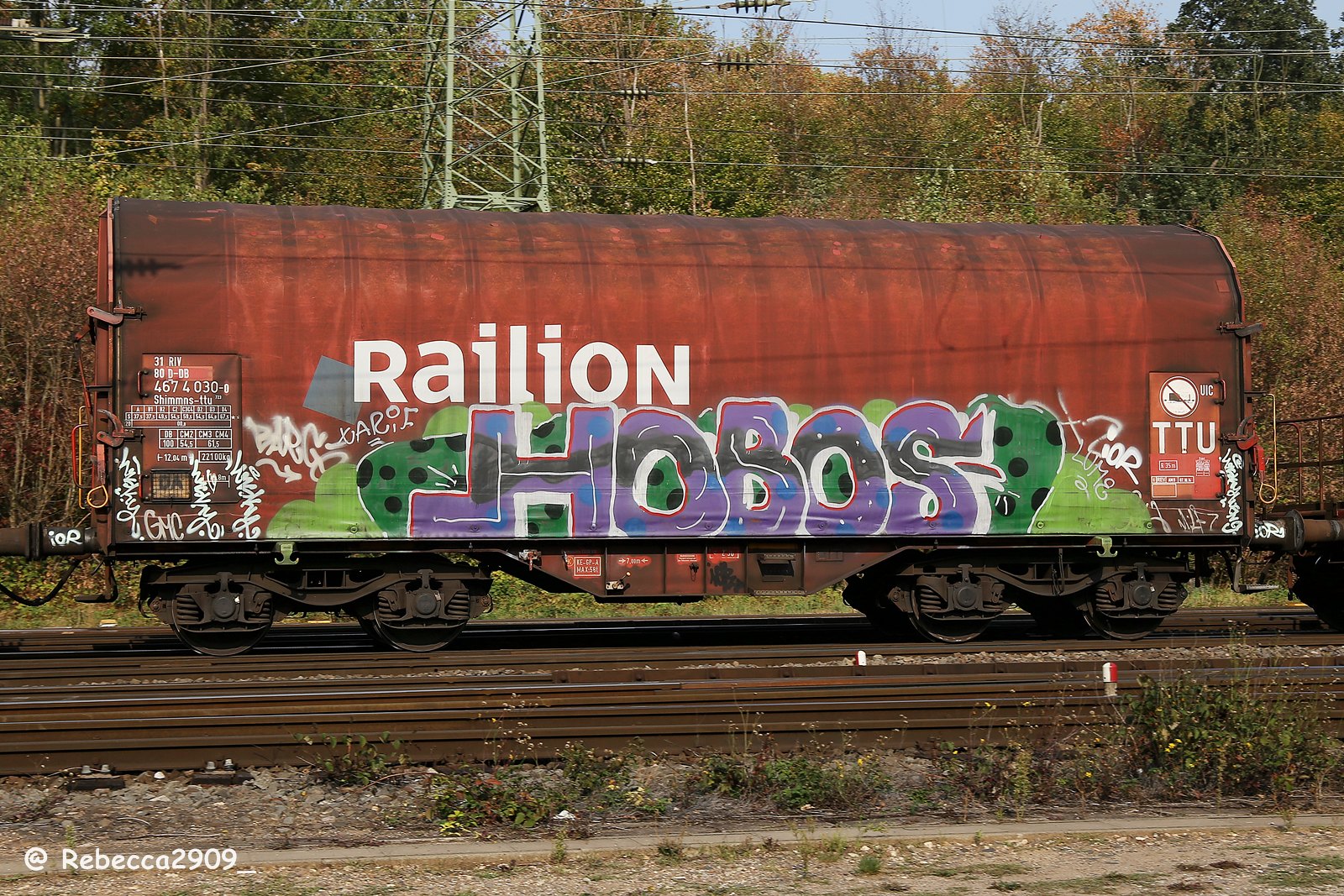The image depicts an old, rusty, red train car with a slightly brown, dirty appearance sitting on train tracks. Prominently displayed in white letters is the word "RAILION" and the abbreviation "TTU" which is positioned near the front. Covering the side of the train is vibrant graffiti, with the word “HOBOS” rendered in colorful bubble letters—primarily purple, black, and blue, with white interiors and outlines. Additional graffiti in green, black, and white is also scrawled across the train, though mostly illegible. The background features numerous power lines stretching between green electrical poles, against a backdrop of trees with leaves that appear to be changing colors. The ground in front of the train consists of dirt with patches of weeds and grass sprouting between the train tracks. The overall scene is framed under a clear blue sky.